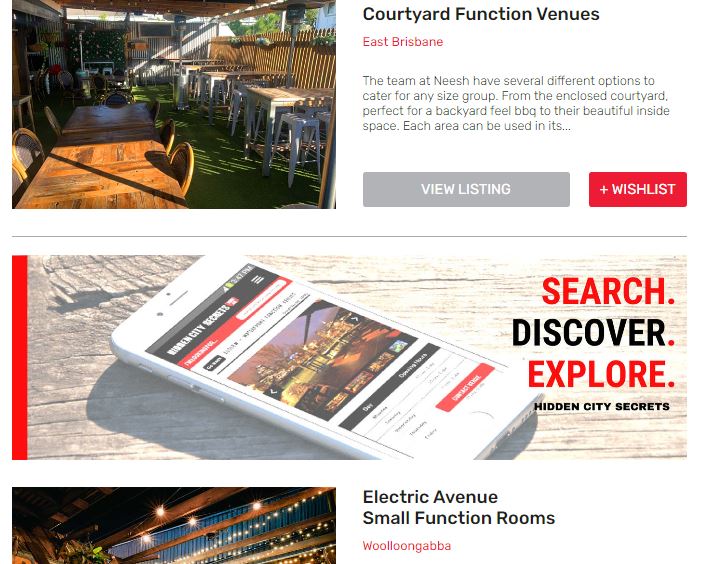In this partial image from what appears to be the Courtyard Function Venues' website, various elements are depicted. The upper portion features a media image showcasing a stack of wooden chairs, each with slatted backs, suggesting either a quaint decorative fence or chair backs, set within what seems to be a Caribbean-inspired setting. Positioned on the left-hand side is a table accompanied by chairs, resting on a floor with a green hue. 

To the right, the text "Courtyard Function Venues" is displayed in red font, just beneath the label "East Brisbane." Below this section, there is a gray rectangle labeled "View Listing" and a red rectangle featuring a "+" symbol alongside the text "Wish List." An adjacent media image of a phone is bordered by a thick red line. Further to the right, the words "Search, Discover, Explore, Hidden City Secrets" are prominently displayed. Continuing downward, another media image is presented with accompanying text on the right that reads "Electric Avenue Small Function Rooms," followed by the location "Woolloongabba."